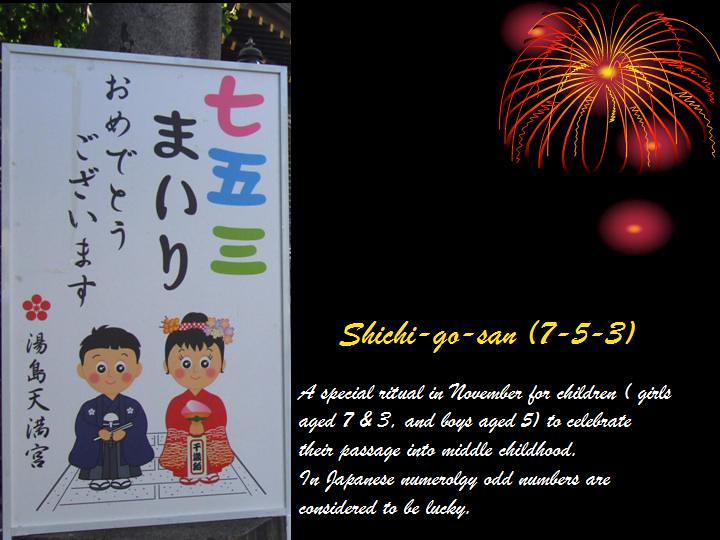The image appears to be a computer-generated black poster designed as an advertisement. On the left side, there is a prominent white sign featuring numerous Asian (likely Japanese) characters. Below this sign, there are cartoonish depictions of a boy and a girl wearing traditional attire; the boy is in a blue robe holding a dish of rice and chopsticks, while the girl dons a red dress with flowers in her hair. On the top right, colorful clipart fireworks in shades of red, yellow, and pink light up the background. Below the fireworks, the text "Shichi-Go-San (7-5-3)" is displayed in yellow. At the bottom of the image, cursive white text explains, "A special ritual in November for children, girls age 7 and 3 and boys age 5, to celebrate their passage into middle childhood. In Japanese numerology, odd numbers are considered to be lucky."